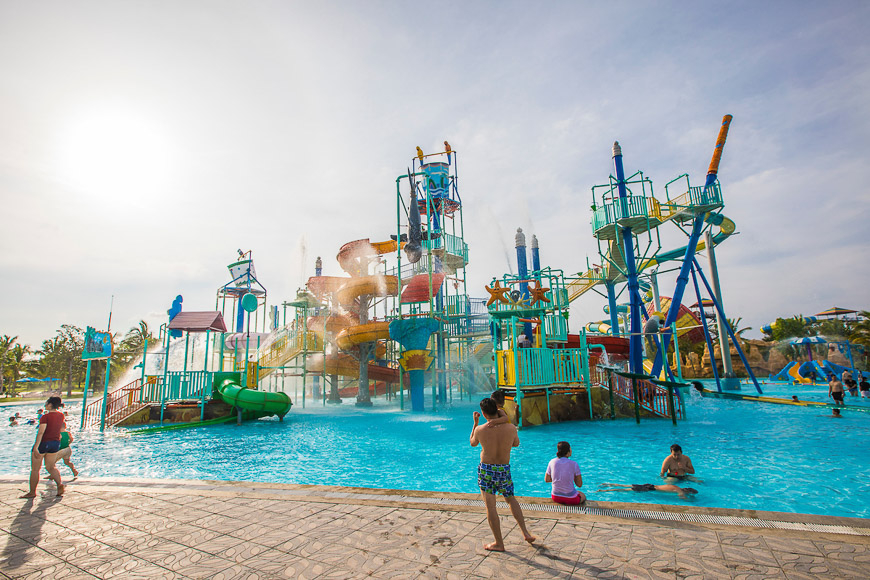In the bright, sunny setting of a bustling water park under a vast blue sky scattered with a few clouds, the picture captures a lively scene. The sun gleams brightly from the left side, illuminating the concrete area below that features a multitude of people. Central to the image is a man in blue and green swimming trunks, holding his child as they look out over the inviting, vibrant blue water. To their left, a woman in a red shirt and blue jean shorts walks hand in hand with her child, about to exit the frame. On the right, a woman in a pink shirt and pink shorts dangles her legs in the water while two men swim nearby.

The water park's centerpiece includes a dazzling array of slides in various colors: a spiraling yellow slide, a smaller green slide, and others. Decorative elements like starfish and intricate designs on the grayish pavement add charm to the scene. Tents and other structures are visible in the background, along with numerous visitors enjoying the attractions. Overall, the picture encapsulates the energetic and joyful atmosphere of a day at the water park.